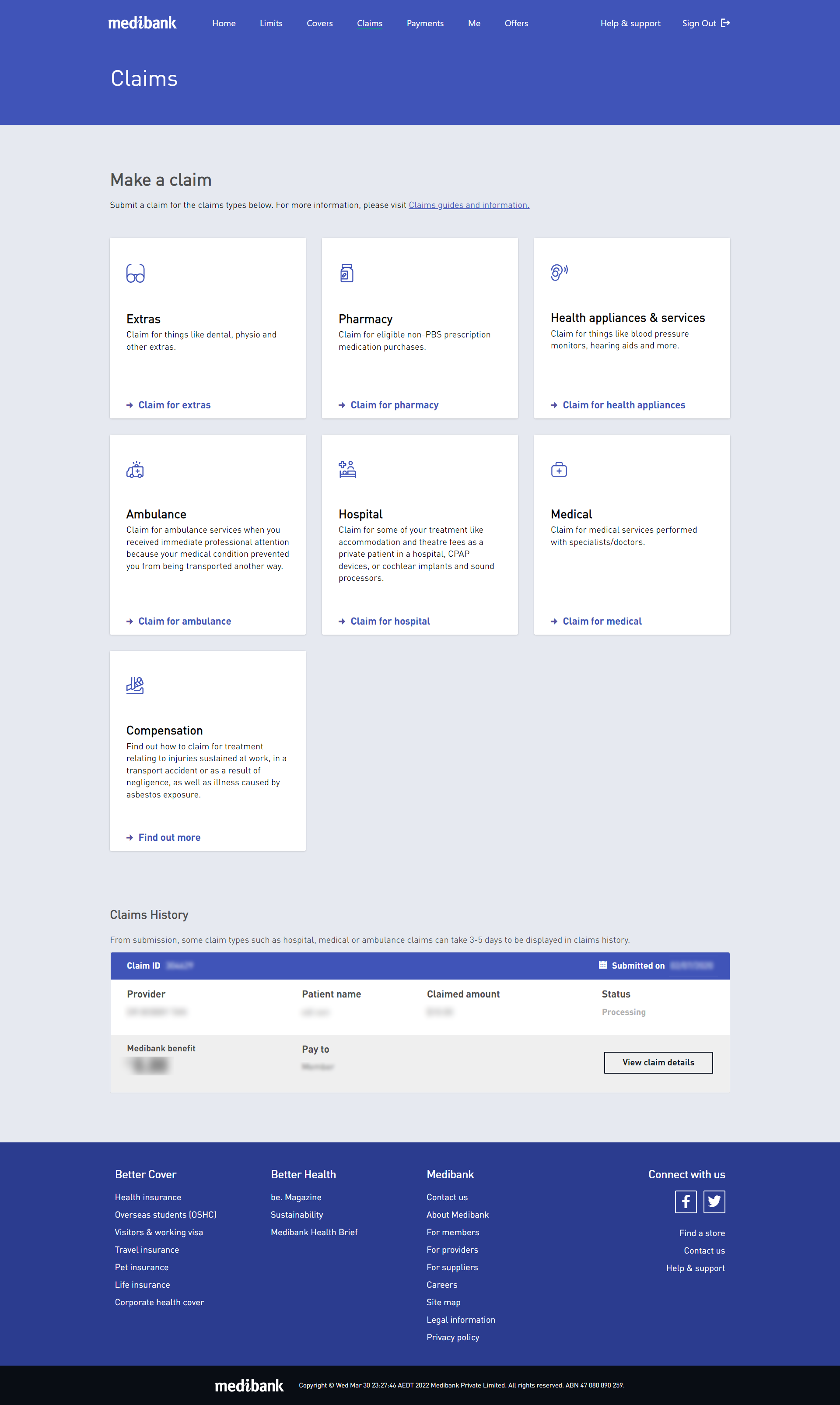This image is a composite screenshot of a Medibank insurance management website, captured on a desktop or laptop in a portrait vertical arrangement to display the entire length of the page. 

At the top, there is a blue banner prominently featuring the Medibank logo in white text. This banner includes navigation buttons labeled: Home, Limits, Covers, Claims, Payments, Me, and Others. Additionally, there are options for Help and Support, and a Sign Out button. 

Directly below this banner, the word "Claims" is displayed in bold white text. The main body of the page is a field offering options to "Make a Claim" or "Submit a Claim." Under these headings, tiles provide various claim categories such as Extras, Pharmacy, Health Appliances and Services, Ambulance, Hospital, Medical, and Compensation.

Further down, a detailed claims history section lists multiple claim IDs, indicating a thorough record of past claims. 

The bottom section of the page has another blue banner containing various helpful links to different sections of the website, including help pages and information resources. It also features social media icons to connect with Medibank on Facebook and Twitter. This screenshot effectively portrays an insurance management website designed to facilitate user navigation and claim submission processes.